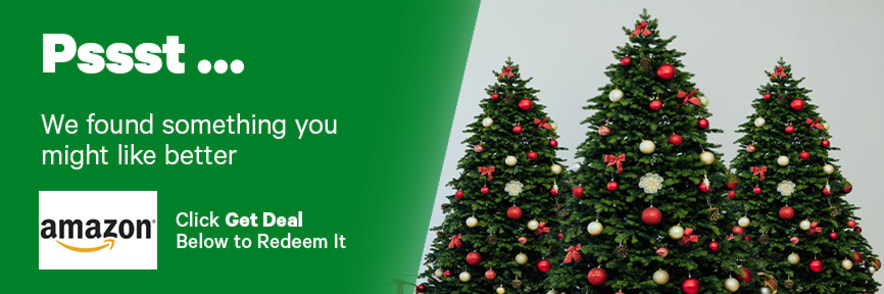Screenshot featuring a gray background. At the top, there is a green square with white text that reads "Pssst... We found something you might like better." Below this is a gray rectangle that contains the Amazon logo accompanied by the text "Click it deal," both in bold. Directly underneath, there's a prompt to redeem the offer.

In the background, against a blue wall, three green Christmas trees are positioned. The center tree appears slightly taller and larger, which may be due to its closer proximity to the viewer. It is adorned with a variety of red and silver ornaments, including several red bows, creating a cohesive festive theme.